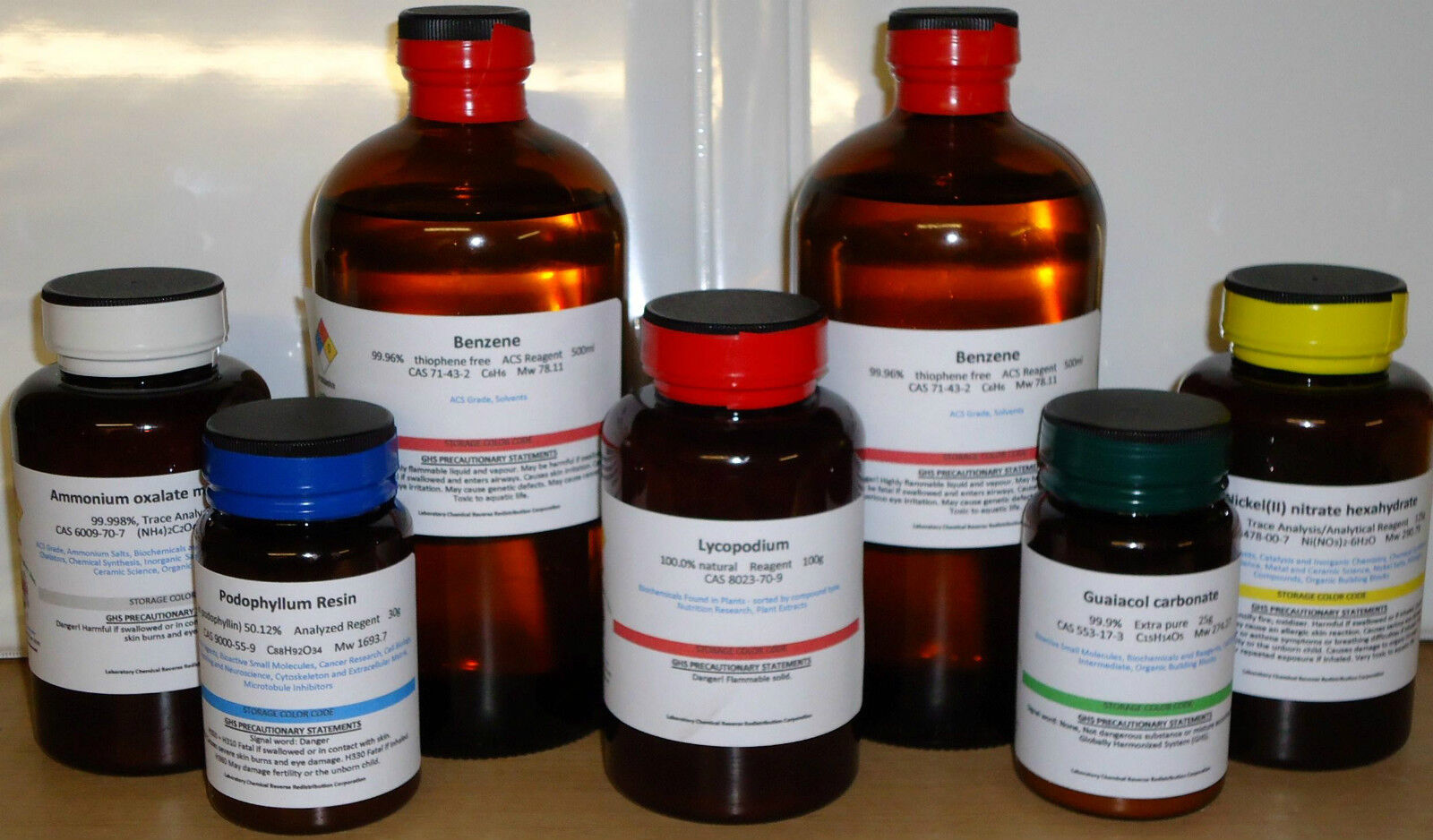The image features seven dark glass bottles of various sizes, all containing chemicals, and situated on a shiny light brown wooden surface against a white painted metallic background. Prominently, there are two large bottles labeled as benzene, each sealed with red safety wrapping, indicating they have not been opened. Among the bottles in the foreground, all also sealed with safety tape of different colors—white, blue, red, green, and yellow—their labels identify them as containing chemicals such as lycopodium, podophyllum resin, ammonium oxalate, nickel nitrate hexahydrate, and guaiacol carbonate. From left to right, the sequence of bottles includes a mid-sized ammonium oxalate bottle, a podophyllum resin bottle, one large benzene bottle, a mid-sized lycopodium bottle in the center, another large benzene bottle, a small guaiacol carbonate bottle, and finally a small nickel nitrate hexahydrate bottle.